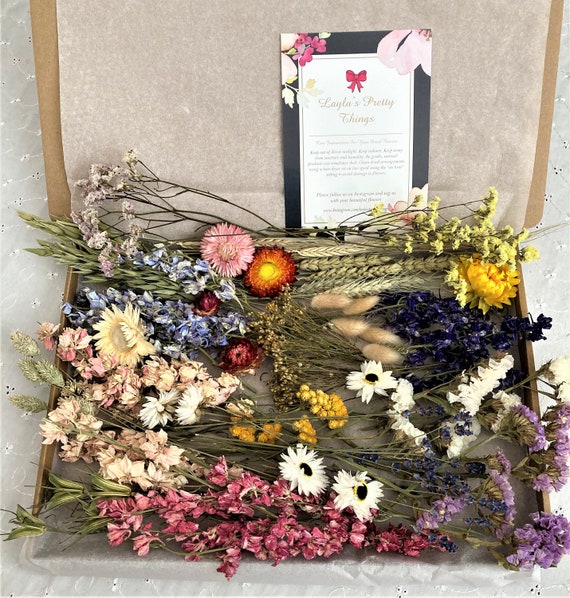The photograph showcases an intricately arranged display of dried flowers in an indoor setting. The flowers are meticulously laid out in a rectangular-shaped box, which is lined with white tissue paper that has a lacy texture. The flowers are still on their stems and feature a vibrant array of colors including pink, purple, ivory, blue, yellow, and even some dark purple or black fuzzy accessory flowers. At the top of the display, tiny wheat stalk-like flowers add a rustic touch. The flowers are layered starting from pink at the base, transitioning to purple and ivory above, with clusters of bright yellow flowers in the center, and ending with blue and additional yellow at the top. 

Above the floral arrangement, the box's lid is open, revealing a note card that reads "Layla's Pretty Things" accompanied by a distinctive pink ribbon. The note card has golden text and is encased in a black edge with a white center, featuring additional unreadable text below the main title. The card also includes decorative elements like a bow tie in the middle and possibly ribbons or floral designs at the top edges. The overall presentation of the box and its contents exudes a charming and elegant floral aesthetic.